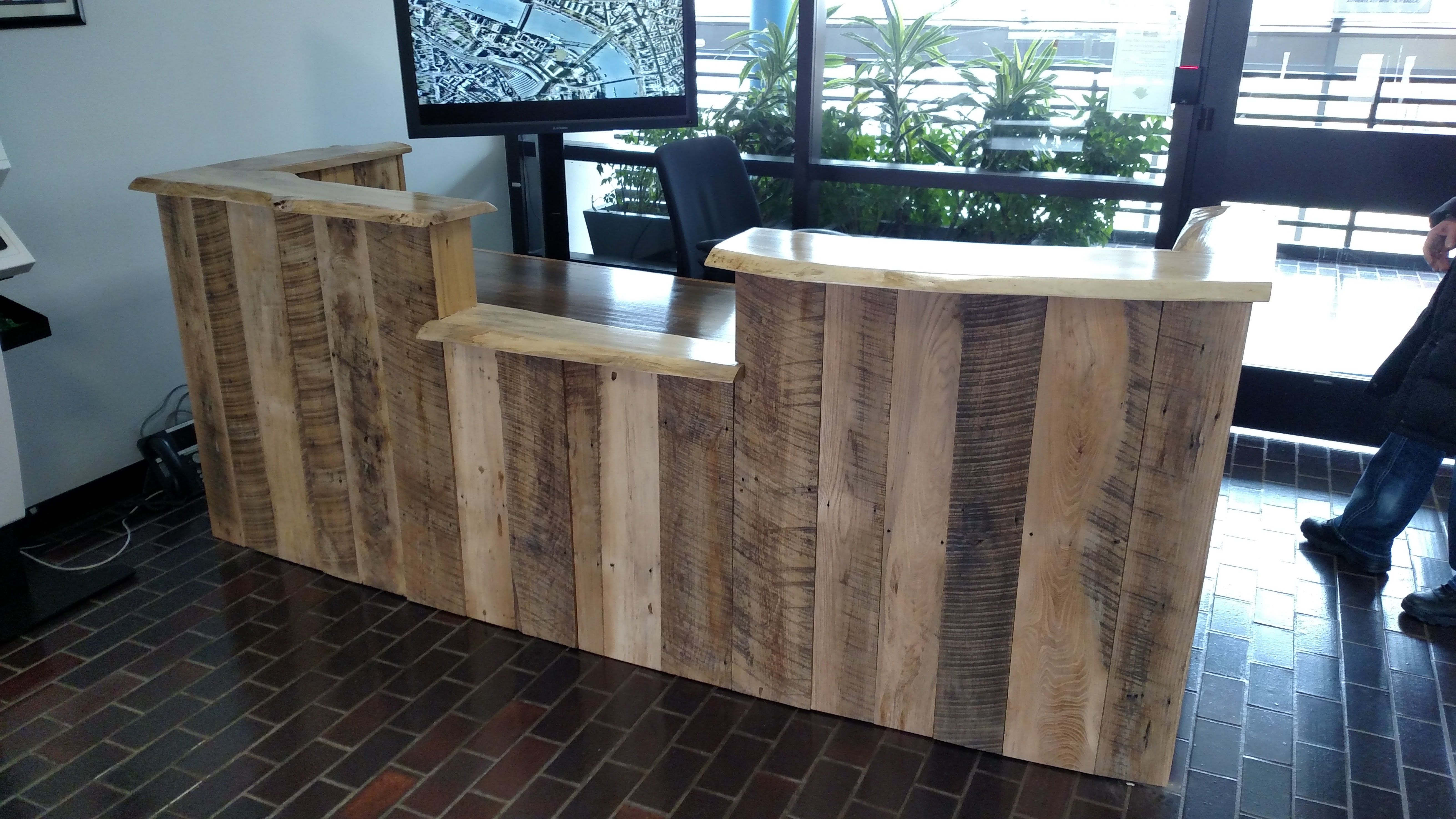The image captures an indoor reception area photographed during the daytime. Dominating the center of the image is a natural wooden desk, prominently featuring vertical or horizontal wooden slats, and a polished, smooth wooden countertop. The design includes raised sides and a lowered center, creating a teller-like spot helpful for interactions, such as exchanging information or handing over documents like licenses or credit cards. 

In front of the desk, the floor is paved with tiles patterned to resemble red and brown bricks, complete with grey grout, adding a rustic charm to the space. Positioned behind the desk is a black office chair, and to its left sits a computer screen or TV on a stand. 

The background is marked by a series of large windows with black frames, allowing ample daylight to illuminate the scene. Through the windows, lush green plants and metal rails can be seen, imbuing the space with a serene, natural ambiance. Additionally, to the upper right of the image, there's a door with window panels. Just within view on the right side are the legs of a person walking, further adding to the liveliness of this well-designed reception area.